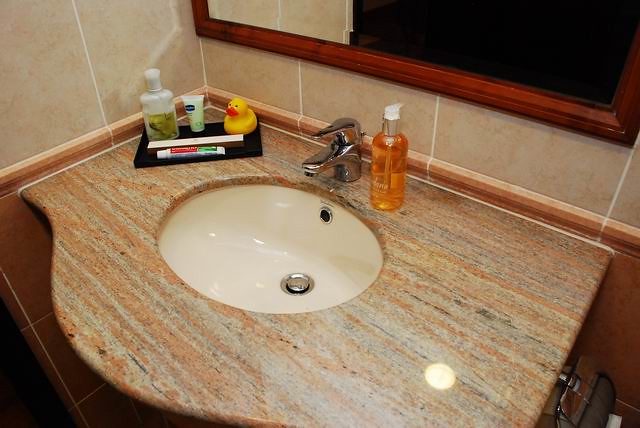In this detailed bathroom image, the sink area commands attention against a backdrop of off-white tiles and a mirror framed by a dark brown wooden border. Positioned in the upper left-hand corner of the sink counter, a charming small rubber duck sits next to a bottle of lotion and a smaller, unidentified bottle, possibly containing dental care items like a toothbrush and toothpaste. On the opposite side, to the right of the stainless steel faucet, stands a clear bottle filled with orange soap. The centrally placed sink is pristine white, set within a countertop that boasts a rich, variegated pattern of browns, tans, blacks, and subtle streaks of blue. Viewed from an angle that suggests the photographer is standing at the right-hand corner of the counter, a toilet paper roll holder is visible, hanging off the right edge of the sink. White grout crisply separates the tiles, completing the orderly and inviting look of this bathroom scene.